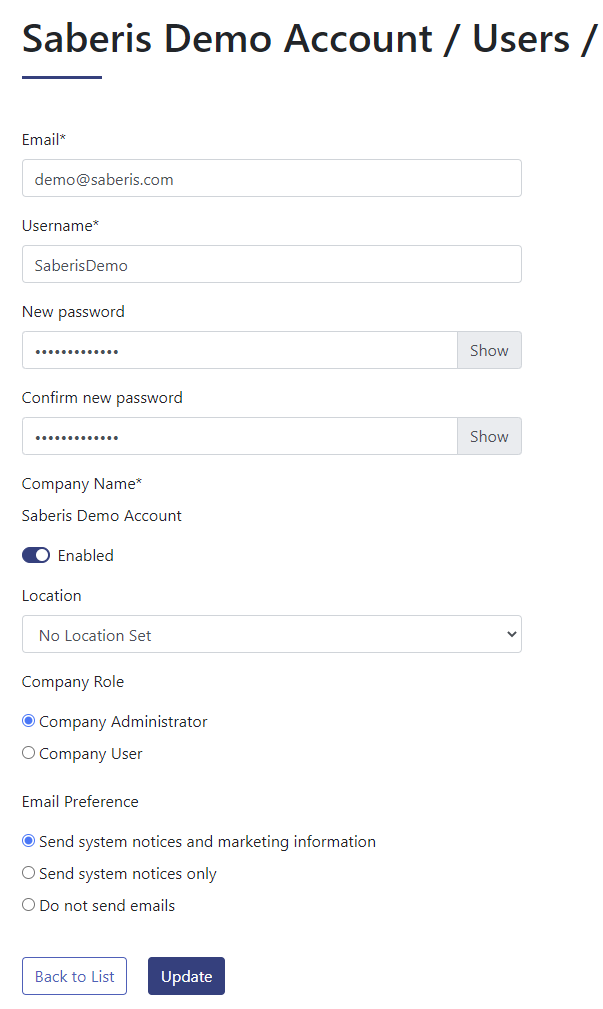The image captures a detailed user interface of a web form titled "Siberius Demo Account" on a completely white background. At the very top, large black text reads "Siberius Demo Account / Users /," with a black line emphasizing the "SABE" in "Siberius."

Directly below, the form is laid out with several fields and labels. The first labeled "Email," marked with an asterisk, has "demo@siberius.com" entered in the field beneath it. Next is the "Username" field, also marked with an asterisk, displaying "Siberius Demo."

Following is a section for setting a new password. It includes fields labeled "New Password" and "Confirm New Password," each with asterisks and containing obscured input represented by asterisks. To the right of both password fields, there are gray "Show" buttons with black text, presumably to reveal the entered passwords.

Below the password fields, the "Company Name" field marked with an asterisk reads "Siberius Demo Account." Next, a toggle switch labeled "Account Status" indicates that the account is enabled, with the switch slid to the right and marked "Enabled."

The "Location" section follows, featuring a drop-down box that currently shows "No action set." Directly below this, the "Company Role" section offers radio buttons for "Company Administrator" and "Company User," with "Company Administrator" selected and highlighted in light blue.

The "Email Preferences" section provides three radio button options: "Send system notices and marketing information," "Send system notices only," and "Do not send emails." The first option is selected.

At the bottom of the form are two buttons for user actions: a white "Back to List" button and a navy blue "Update" button.